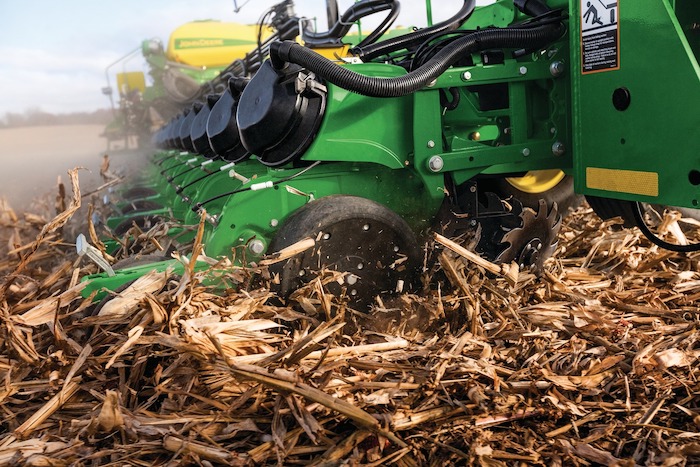In this action shot taken on a vast farmland, we see a large, green, and yellow farm machine, likely a wood chipper or similar agricultural equipment manufactured by John Deere. The machine, adorned with multiple wheels and black hoses connected to its various components, is actively in operation. It appears to be moving forward through a field under a diffuse blue sky, which is partially obscured by dust and smoke generated by the machine’s activity. In the foreground, wood chips and dried plant material are being vigorously processed and scattered by the machine's numerous blades, while the recognizable John Deere logo can be seen in a blurred background. The machine’s powerful performance suggests it's being used at a fast pace, presumably in a large field, highlighting its efficiency and possibly serving as an advertisement for John Deere's robust farming machinery.